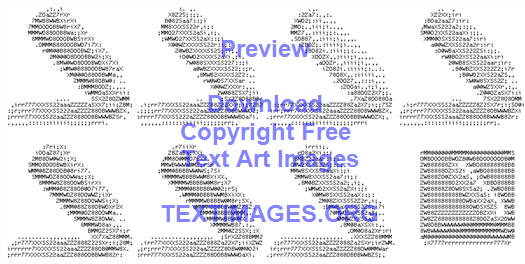This image is a text art creation composed entirely of black and white dot patterns. It features two rows of identical, V-shaped designs, each construct resembling a sideways view of a microphone propped up. Superimposed over these rows are the words "PREVIEW," "DOWNLOAD," "COPYRIGHT-FREE," "TEXT ART IMAGES," and "TEXTIMAGES.ORG," all displayed in purplish-blue ink. The dots meticulously form the visuals, and in the bottom right corner, there is an enclosed square containing a smaller version of the dot image, illustrating intricate detail and precision in the text art format.